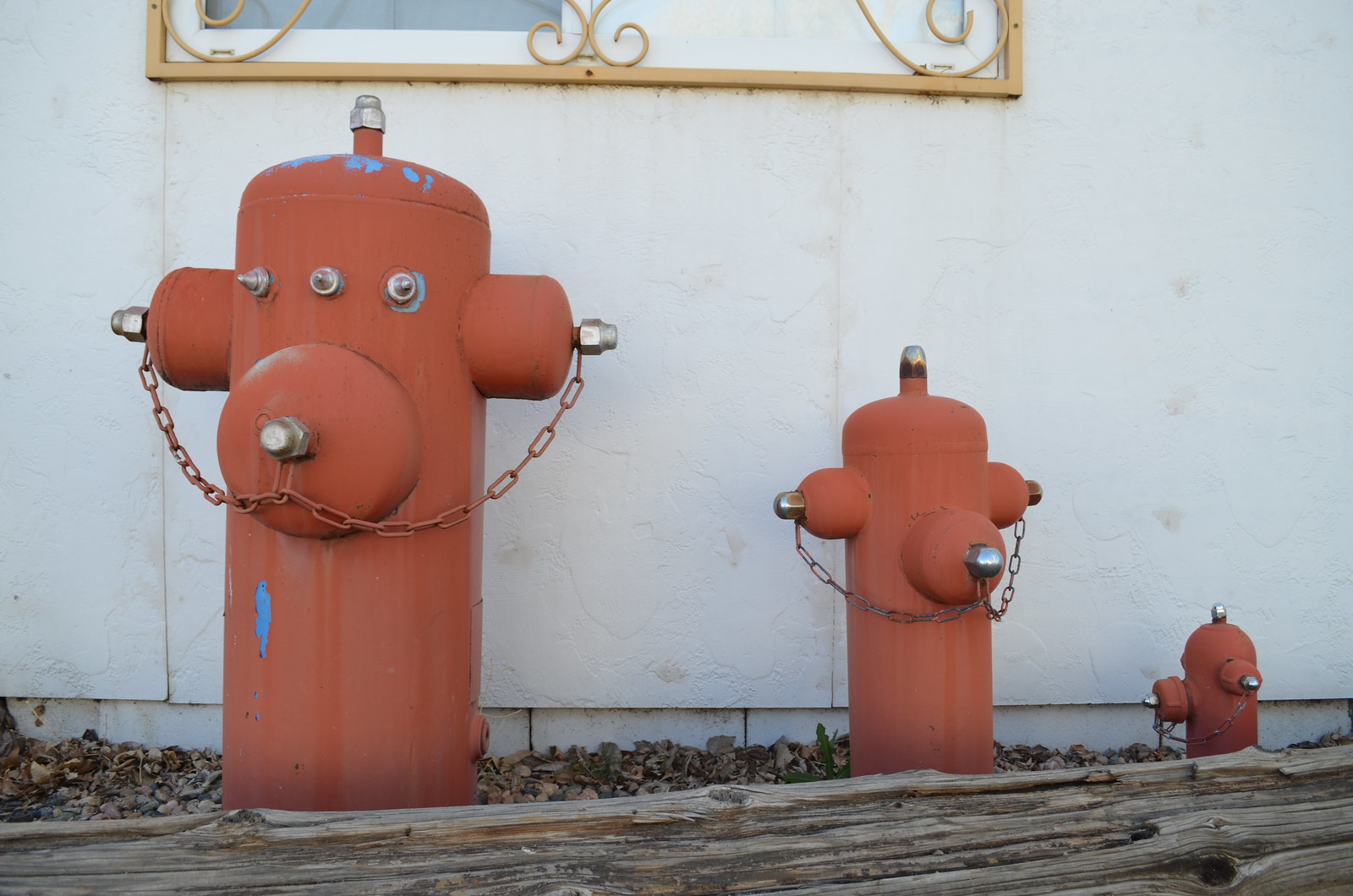The image features three red fire hydrants of varying sizes placed side by side in front of a white building. The largest hydrant, positioned on the left, stands about waist height and shows signs of paint flaking, revealing a blue undercoat beneath the faded red surface. It has a bolt on top and three bolts in the center, with chains connecting the bolts in a characteristic fire hydrant fashion. The middle hydrant, which is about half the size of the largest, also has three cap openings and a chain. The smallest hydrant, standing on the right and roughly 15 inches tall, appears to have one missing side cap and is slightly turned to its left. All three hydrants are set against a backdrop of gravel and mulch, with a rough piece of driftwood or wooden walkway in front. Above the hydrants, the bottom part of a brass-framed window with a gold gate is visible. The wall behind them is white with brown dirt marks, completing the charming yet slightly surreal exterior scene.